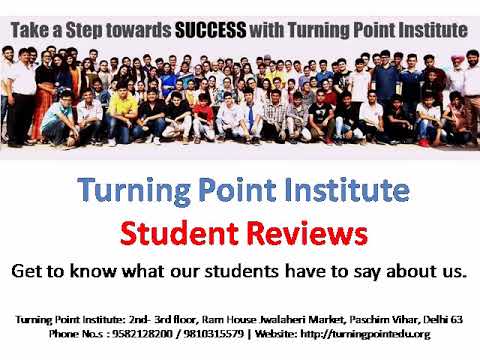This is an advertisement poster for the Turning Point Institute. The top portion features a light blue background with a panoramic photo of approximately 60-100 people arranged in rows, from kneeling to standing. Above the image, the bold black text reads "Take a Step Towards Success with Turning Point Institute," with "SUCCESS" notably in all caps. The middle section of the poster transitions to a white background, prominently displaying "Turning Point Institute" in large blue Arial font. Directly beneath it, "Student Reviews" is written in red font. Below this, in black letters, it reads, "Get to know what our students have to say about us." The bottom section of the poster provides detailed contact information in smaller black text, including the address: Turning Point Institute, Second & Third Floor, Ram House, Jalwalari Market, Pershim Fault, Valdir Del Hai 63. It also lists two phone numbers: 989582128200 and 9810315579, along with the website: http://turningpointedu.org.